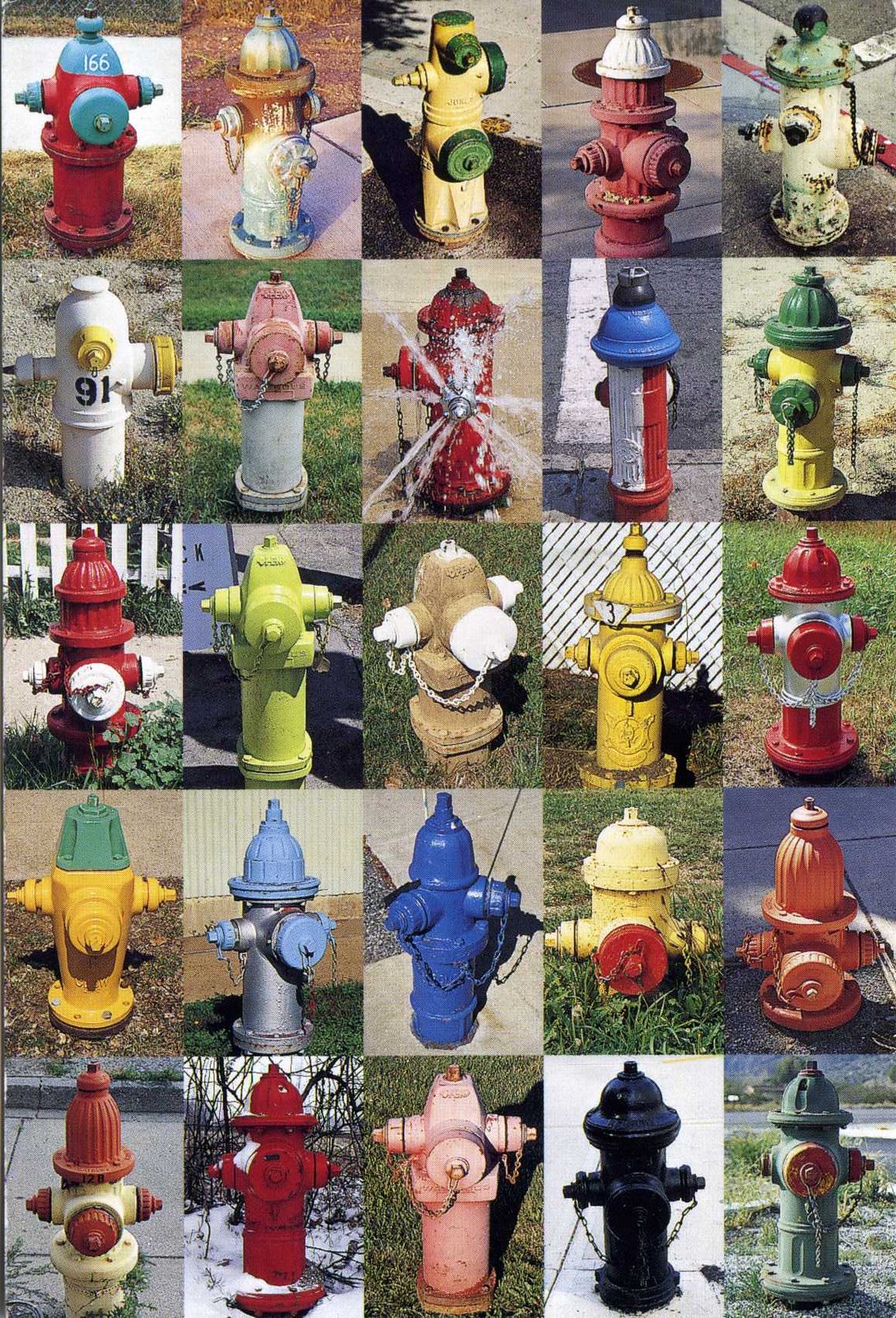This is a detailed collage composed of 25 individual images of fire hydrants, arranged in a 5x5 grid. Each fire hydrant is captured in its own distinctive style and vibrant color, featuring a broad spectrum of hues and designs. Notably, these hydrants range from traditional red and yellow to more eclectic combinations like blue and silver, black and green, and pastel colors. Midway through the second row is an eye-catching hydrant spraying water in all directions. Several hydrants in the third row are adorned with chains hanging from either side. These hydrants are situated in diverse settings, from city streets to garden landscapes. The backgrounds of each image vary, showcasing fences, cement, grass, and various decorative elements. Some hydrants are repainted or decorated, including colors such as bronze paired with light blue, dark green and yellow, red and white, pastel yellows, and even a statue of liberty green. There's also a unique terra-cotta-colored hydrant and others with gleaming finishes like silver and gold accents. This collage transforms functional urban fixtures into a colorful, diverse visual celebration.